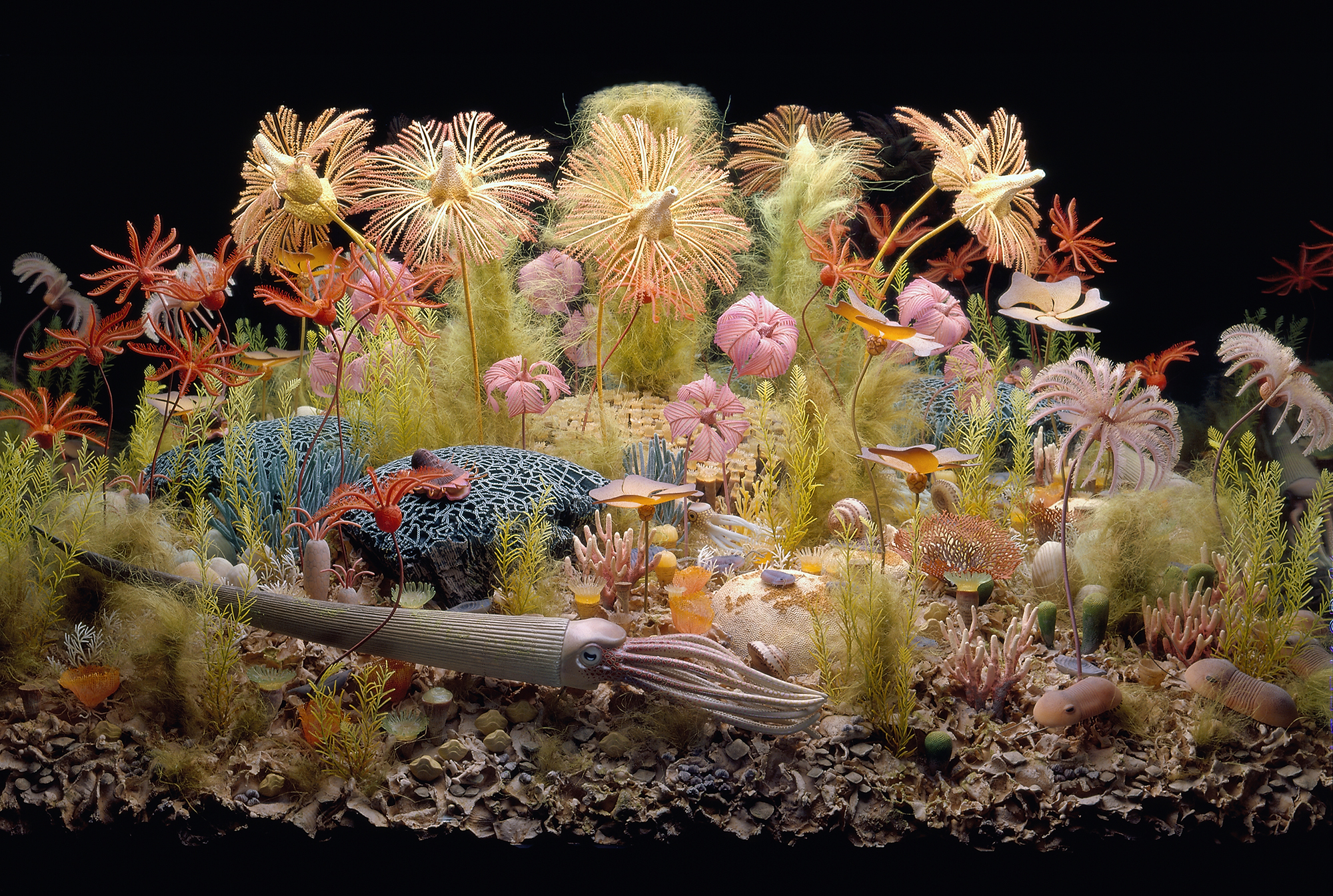The image depicts a rectangular, shadow box-like display that is wider than it is tall, featuring an elaborate ocean floor scene. The background is pitch black at both the top and bottom, creating a dramatic contrast to the vibrant elements in the foreground. The scene is set on a rocky, brown ocean floor and showcases a variety of marine life. Central to the image is a gray stingray or some other swimming animal. The underwater vegetation includes an array of colorful plants, with prominent yellow, pink, and cream-colored flowers. Additionally, there are corally pink-orange flowers with long stems and pink flowers with umbrella-like petals. Various pieces of blue and green coral dot the scene, along with some shells. A white squid and an octopus, partly hidden in a long tube at the bottom, add to the aquatic diversity. The overall aesthetic is rich in color, featuring hues such as pink, red, brown, yellow, orange, blue, black, lime, and a touch of off-color red. This image could either be a well-crafted photograph of an aquarium or an AI-generated visual, though it contains no text.